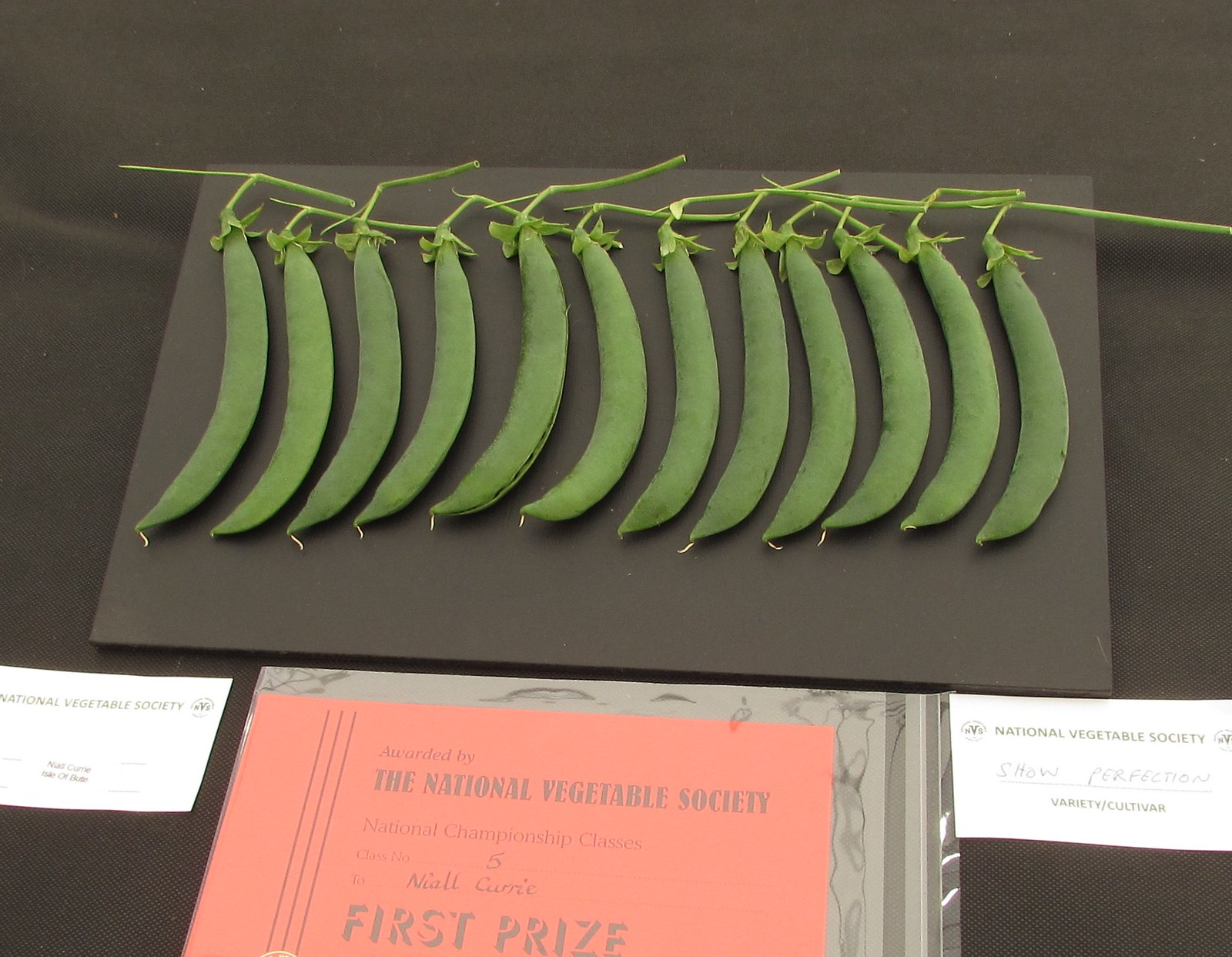The photograph depicts a pristinely arranged display of green sugar snap peas or possibly snow peas. These vegetables, which are long and undamaged, are placed neatly in a single-file line on a black rectangular board. Two cards are present; a bright orange card below declares the award from the National Vegetable Society National Championship Classes, stating "First Prize," while another tag on the left specifies "National Vegetable Society Variety Cultivar Show Perfection." The visually appealing and fresh-looking peas, unpeeled and with their light green stems attached, suggest recent harvest and excellent quality.